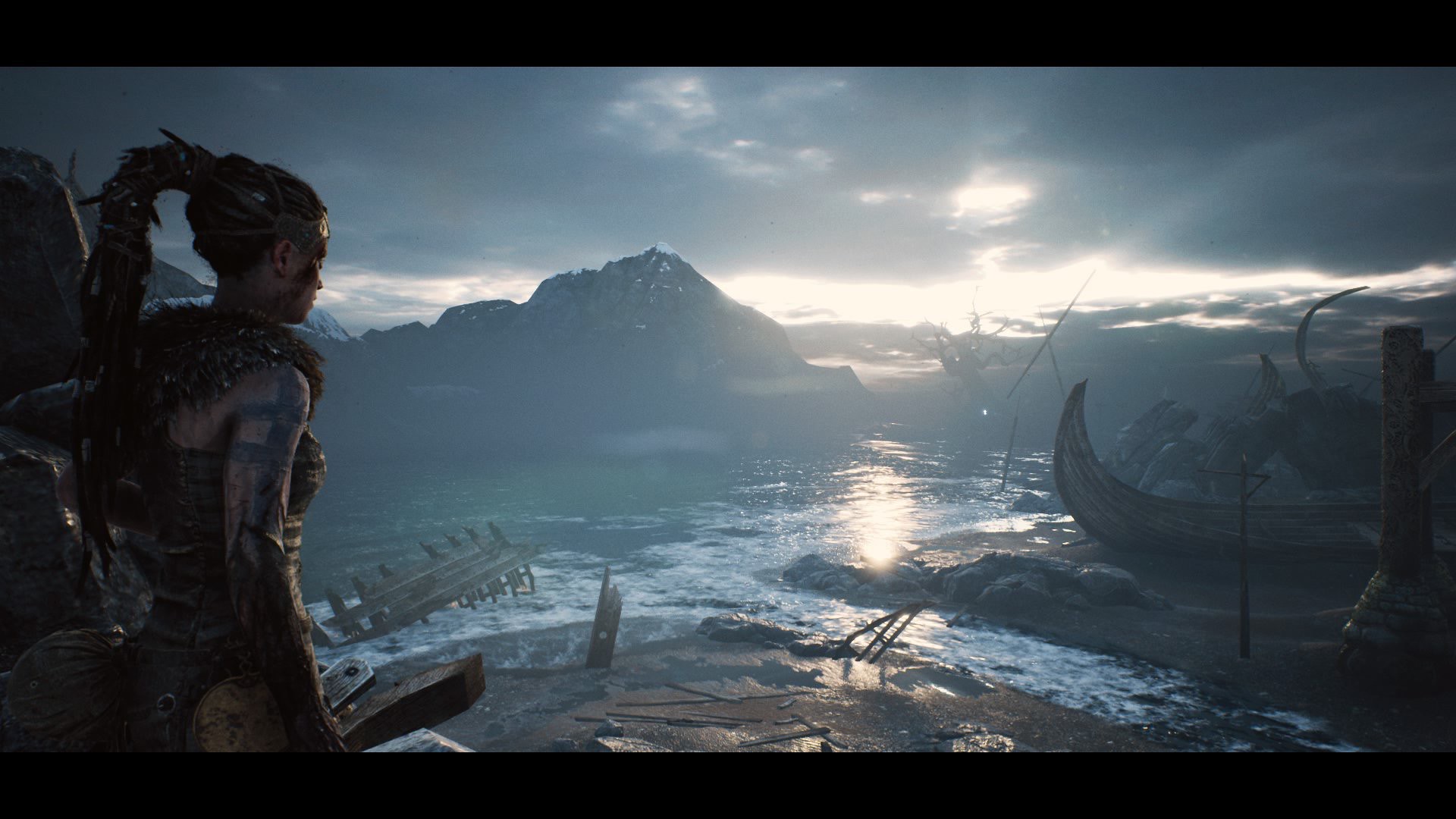The image is a dramatic scene from the critically acclaimed video game "Hellblade: Senua's Sacrifice" by Ninja Theory. The main character, Senua, stands on the edge of a cliff, looking off into the distance where the sun is breaking through a cloudy sky, casting rays of light. She wears tight-fitting, somewhat skimpy armor that runs around her neck, down her back, and chest, complemented by tattoos and braids on the back of her head. Her bare arms and the sword in her hand suggest readiness for battle. Below her, a body of water stretches out, flanked by distant mountains. On the water, there are two vessels: a smaller boat with people rowing on the left, and a larger ship on the right. The scene is imbued with a sense of foreboding, enhanced by scattered debris, including pieces of wood, in the foreground, which hint at past destruction.